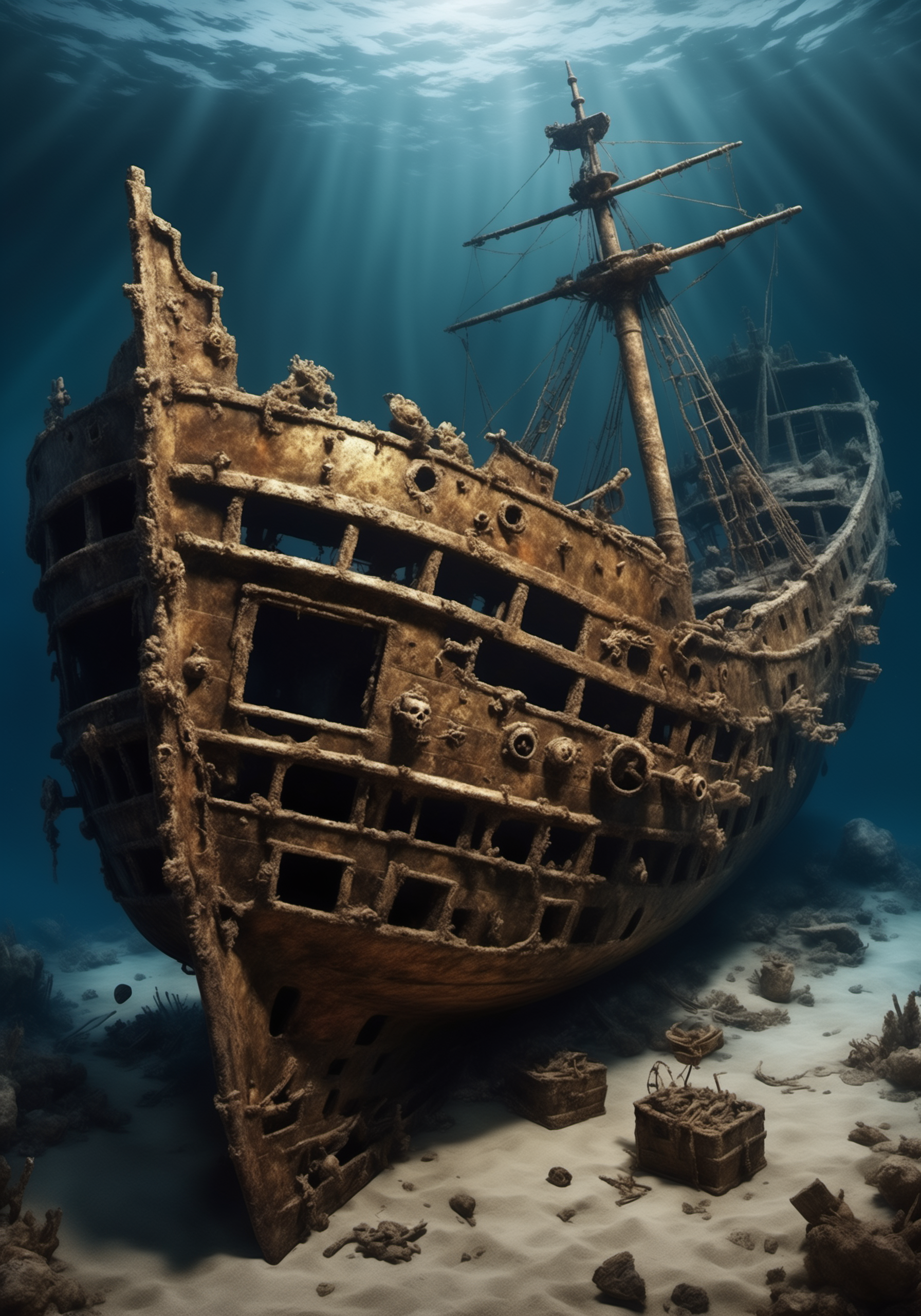The image is a detailed painting depicting an underwater scene featuring the wreckage of an ancient wooden ship resting on the sandy bottom of the sea. The ship, brown and eroded with age, is in a state of severe decay, its structure largely crumbled and falling apart. Surrounding the wreck, the sand is interspersed with rocks and triangular-shaped baskets filled with unspecified items, also in varying shades of brown. Among the scattered debris on the sea floor, a human skull is visible, adding an eerie touch to the scene. The water around the wreck is a soft blue, suggesting shallow depths, and rays of sunlight penetrate from above, casting an ethereal glow on the sunken vessel and illuminating the underwater tableau.